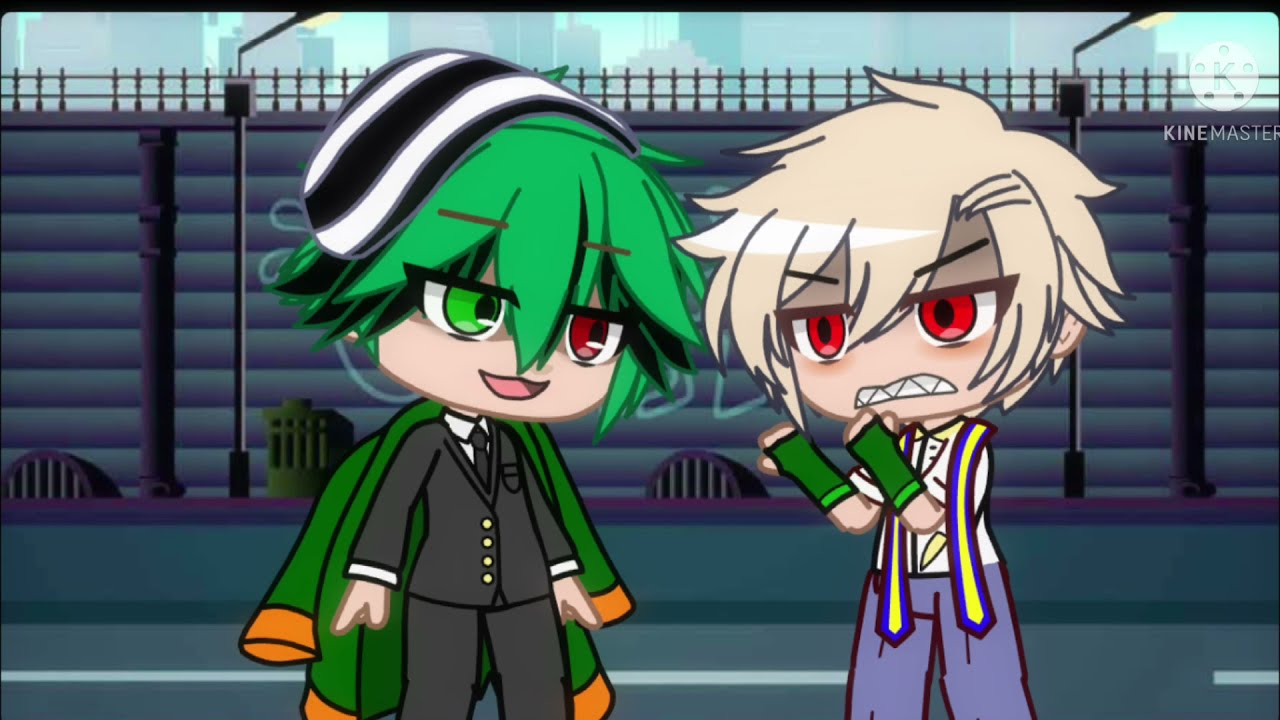In this vibrant, anime-style cartoon image, two central human figures take up most of the frame, set against a backdrop featuring a high gray wall with a railing and a street visible at the bottom. In the upper right-hand corner, there's a logo that says "KineMaster" within a white circle. 

The figure on the left has distinctive green hair and heterochromatic eyes—one green and one red. They are wearing a formal black suit paired with a black tie, partially covered by a green coat with orange cuffs draped over their shoulders. Atop their head, they wear a black and white knit cap. This character’s mouth is open, displaying an expression that adds to the overall scene's tension.

Facing them is a blonde-haired character with a combative stance, fists raised as if ready to fight. This character has striking red eyes and an angry expression, showing off aggressive teeth. They are dressed in blue pants held up by yellow and blue suspenders over a white shirt, with green sleeves over their arms. 

The image artistically captures a moment of confrontation between these two vividly detailed characters, set in a seemingly urban area hinted at by the structure and street behind them.